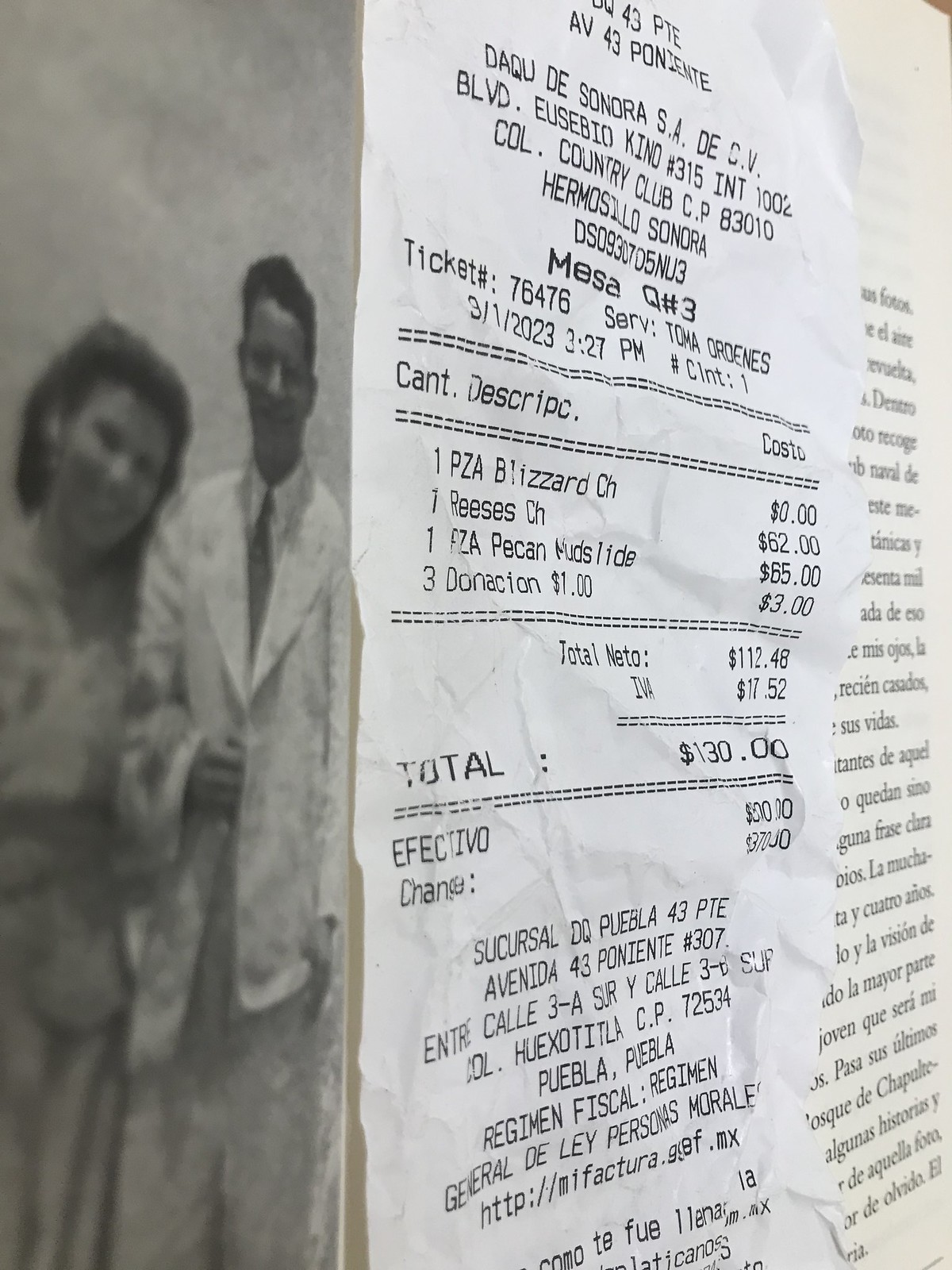The photograph captures an open book with text in Spanish on the right page and a black-and-white image on the left side displaying a man in a white suit and a woman with curly hair in a dress, likely from the 1950s. Placed prominently in the foreground is a white restaurant receipt, also predominantly in Spanish, displaying the name "Dacua de Sondra" which hints at a Hispanic location. The receipt, which details a purchase including items like a PZA blizzard, a Reese's dessert, a pecan mudslide, and three $1 donations, totals $117.48 before tax and $130 after tax. Furthermore, it features essential information such as the address, the server's name, the date, time, and a website at the bottom.